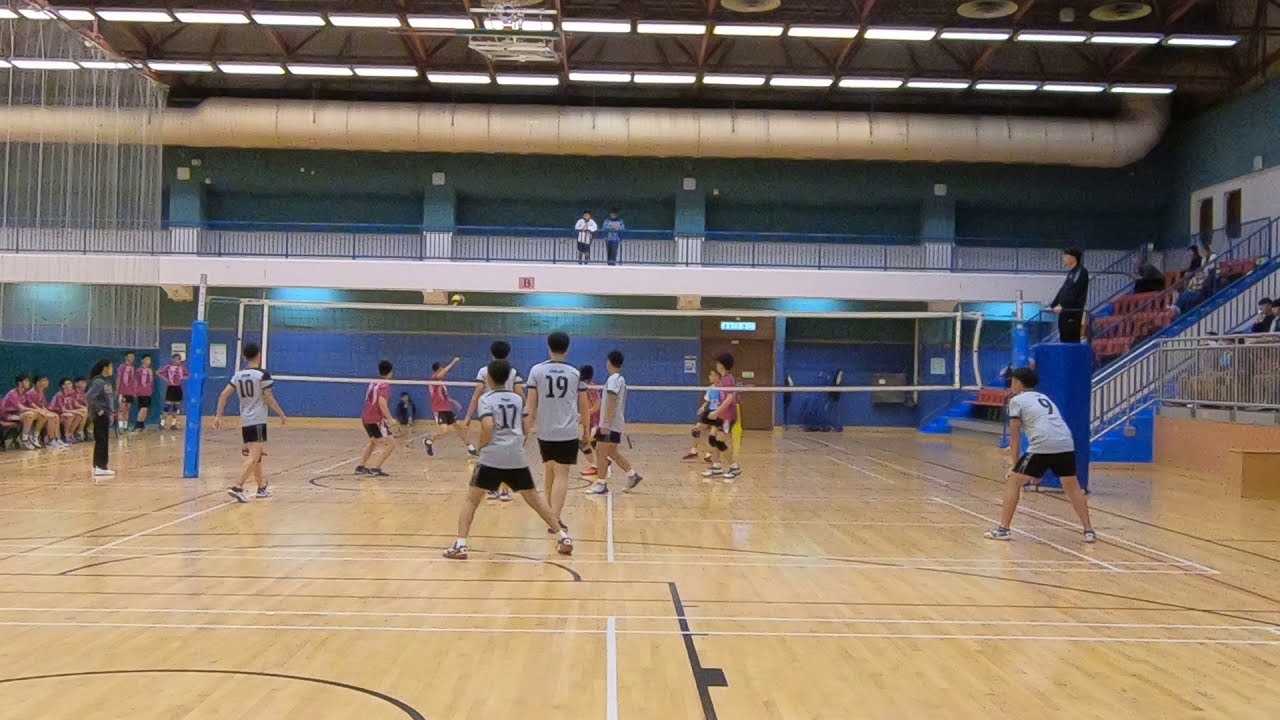This detailed photograph captures the intense action of an indoor volleyball game set in a gymnasium with hardwood floors, likely in Asia given the appearances of the players. The foreground showcases a team in light gray short-sleeved jerseys with black shorts and black numbers on their backs orchestrating their positions, particularly with players numbered 11, 17, 19, and 9 visible from left to right. They are matched against a team in rose-pink jerseys and black shorts, discernible in the mid-ground and background, partially obscured but clearly identifiable by their distinct uniforms and occasional knee pads.

The game's net, white in color, stretches across, supported by blue posts at either end. To the right of the image stands the referee, dressed in a black suit, overseeing the game from atop a blue spongy stand. Stadium seating lines the left side of the court, where additional players from the rose-pink team can be seen waiting. Similarly, empty red bleachers with blue railings on the right hint at a potential practice game, though a few onlookers can be seen scattered around, including some on a second-level balcony.

The gymnasium's ceiling is adorned with fluorescent lighting and an expansive industrial pipe, contributing to an industrial yet structured environment. The scene epitomizes the dynamic and focused nature of a volleyball game, marked by the keen attention of the players and the few spectators scattered throughout the gym.